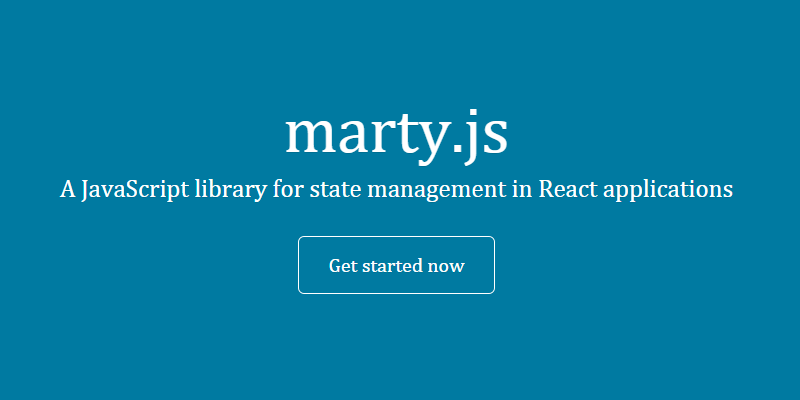"A promotional banner for Marty.js, a JavaScript library designed for efficient state management in React applications. The banner features a sleek blue background and crisp white text, inviting developers to 'Get started now.' The clean design and encouraging call to action evoke a sense of readiness and ease, enticing viewers to dive into using Marty.js for their next React project."